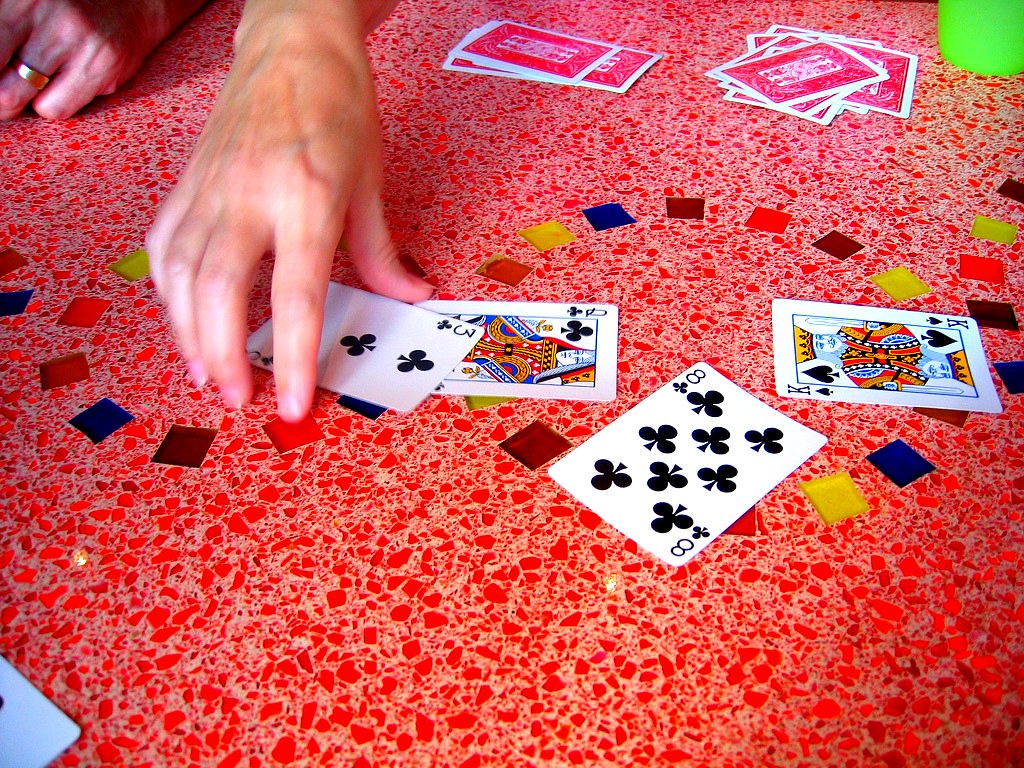The image showcases an intricately designed casino or card table, featuring a vivid red surface with a pattern reminiscent of tiles or stained glass. In the top left corner, a player's hand adorned with a gold wedding band is visible, while another hand reaches for the three of clubs positioned at the table's center. The topmost area displays two piles of cards that seem to be discard piles, although the exact quantity is indeterminate. 

Below the three of clubs lies the queen of clubs, while to the right of these cards are the eight of clubs and the king of spades, contributing to a total of four face-up cards. In the bottom left corner, only the edge of another face-up card can be seen; its details are unclear. In the top right corner, a neon green object is partially visible, though its nature remains mysterious. 

The table itself is embellished with circular designs composed of multicolored squares, including red, yellow, blue, and black, upon which the cards rest. These colorful squares might serve a decorative purpose or have a specific function in the game.